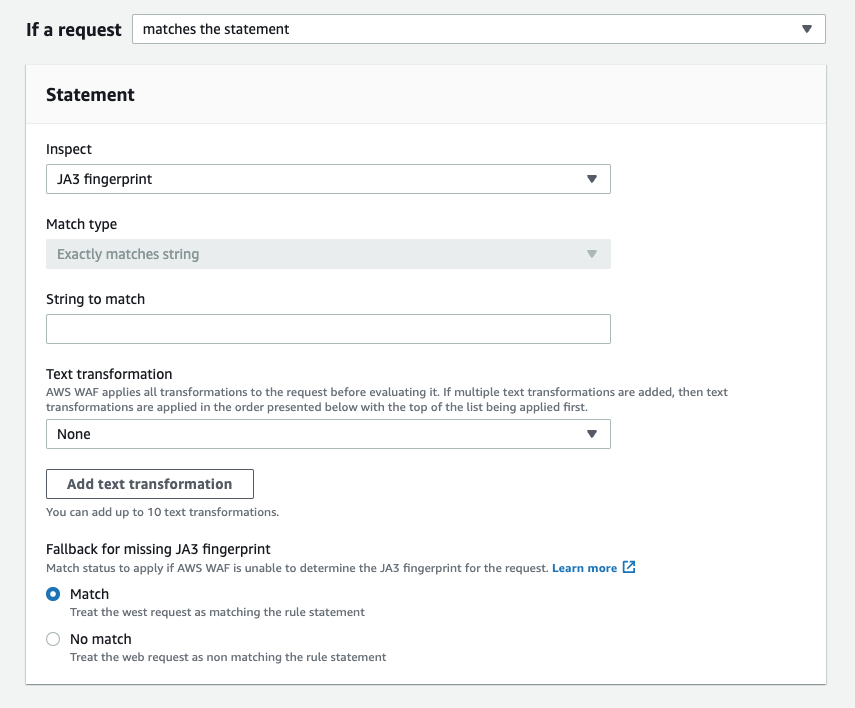The image appears to be a screenshot of a web interface. Dominated by a white background with black text, it is encompassed by a gray border that gives the image a square shape. 

In the top left corner of the interface, there is a section labeled, "If a request," followed by a large input bar to type in text. Adjacent to the input bar is the continuation of the statement, "matches the statement."

Below this, a white box area is segmented further. The first line within this area reads, "Statement," followed by the term "Inspect." Directly beneath this, a box is labeled, "JA3 fingerprint." 

Continuing down, another label reads, "Match type," next to a gray box that states, "Exactly matches string."

The subsequent section is labeled, "String to match," accompanied by a blank input box. Following this, the text, "Text transformation," appears alongside some small black text.

Another box below this section has the word "None" pre-filled inside it. 

Further down is a smaller box labeled, "Add text transformation," with the instruction, "Add up to 10 text transformations," displayed beneath it.

At the bottom left, there is a sentence indicating a fallback mechanism: "Fallback for missing JA3 fingerprint. Match status to apply if ASFWWFAF is unable to determine the JA3 fingerprint."

Lastly, an option labeled "Match" is selected, and underneath, it states, "Treat the request as matching the rule statement."